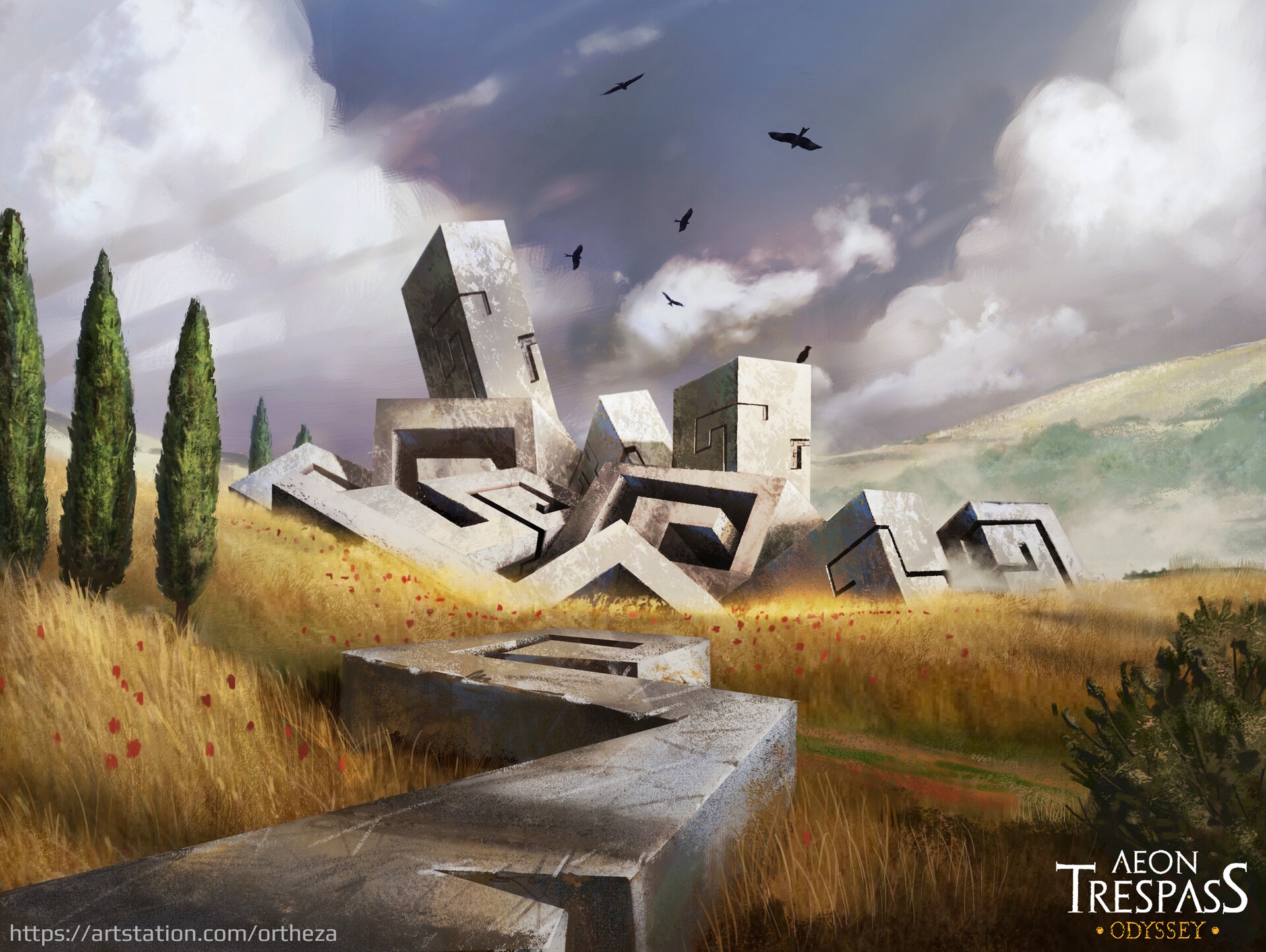The image showcases a desolate, meadowy landscape with tall, dead grass interspersed with red flowers. On both sides of the image are small green trees and bushes, with more trees visible further back. The sky is filled with fluffy, cumulus clouds, creating a stark backdrop to the scene. Dominating the center are various gray, stone-like structures, possibly ancient symbols or fallen modern buildings, many of which have distinct lines carved into them. Some carvings are deep while others are shallow, adding to the mysterious atmosphere. Among these structures, birds are seen flying overhead, evoking a sense of abandonment and decay. At the bottom of the image, the text reads "Aeon Trespass Odyssey" in white and gold, suggesting it is an advertisement for a game. The bottom left corner features a website link, "https://artstation.com/orthiza." Overall, the image conveys a bleak yet intriguing environment, with the presence of life amidst ruin hinting at hidden stories and mysteries.